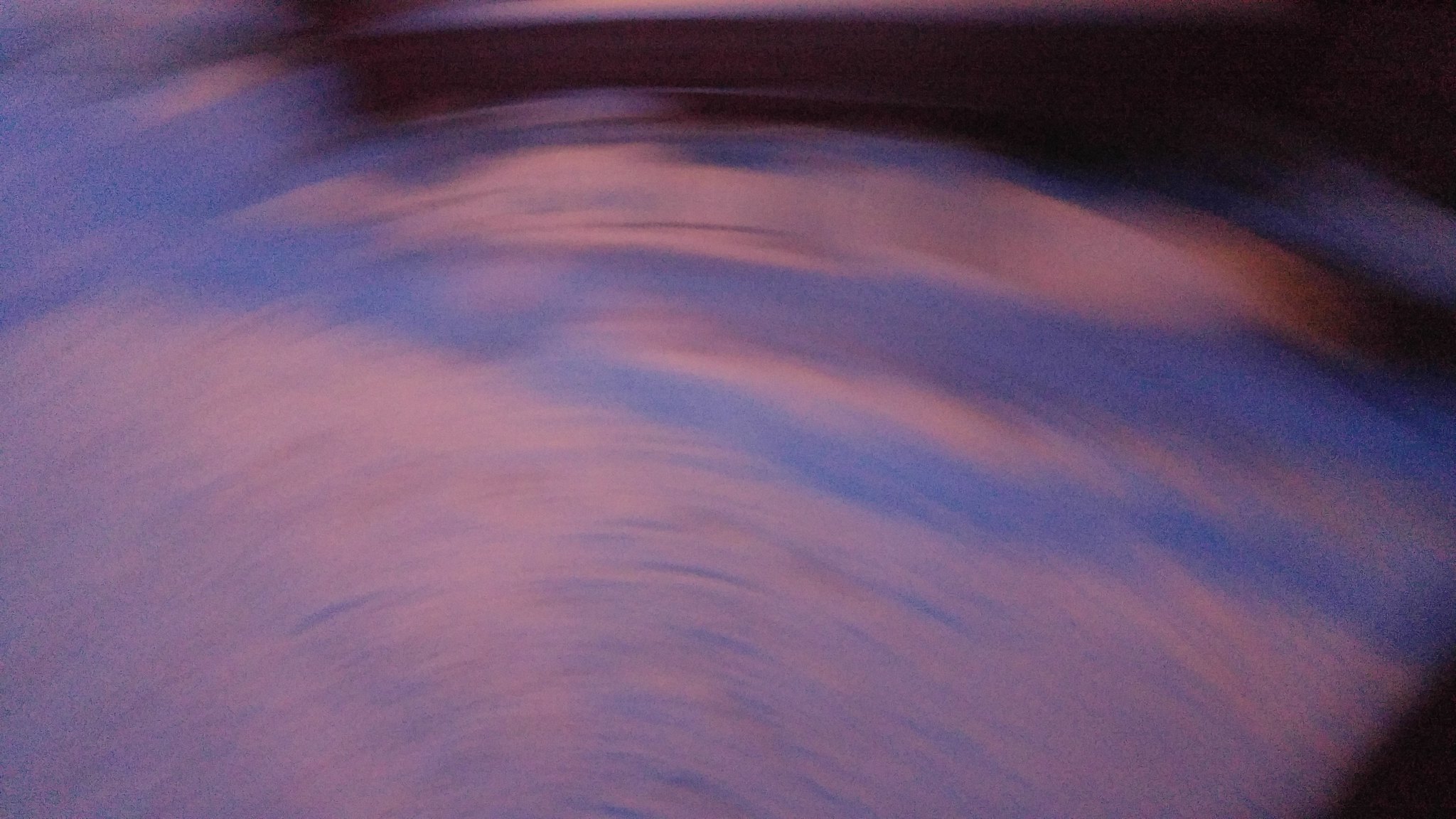The image showcases a blur of colors, likely a result of the photograph being taken in extreme motion, either by the photographer spinning or the camera swinging in a circle. Dominating the scene is a swirl of light and dark blue, intermixed with pink-tinged fluffy clouds, creating a whirlwind effect. Toward the outer edges, darker hues of blue, black, and gray frame the swirl. The image is so blurred that it's open to interpretation, with some perceiving it as either a sandy area bathed in pink and orange reflective light or as a close-up of a bedsheet illuminated by sunlight streaming through a window, casting intricate shadows. The overall effect is an indistinguishable yet fascinating blend of colors and shapes, embodying an abstract and captivating aura.